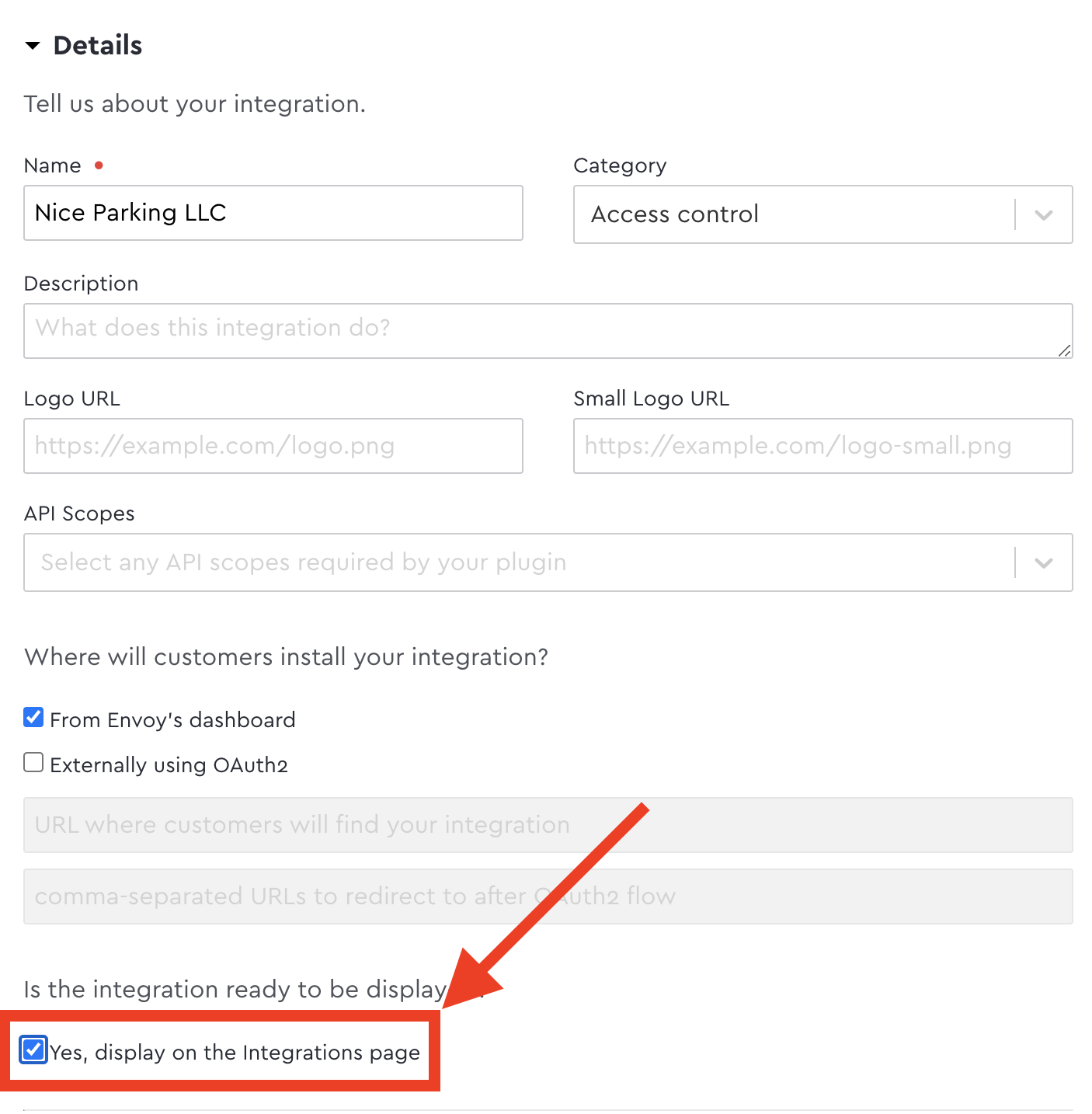The image depicts the admin section of a website's integration management page. Various fields and options are available for configuring an integration. Key elements of the section include:

1. **Integration Details:**
   - **Name:** Input field to specify the integration's name.
   - **Category:** Dropdown menu for selecting the integration category, labeled "Nice Parking, LLC."

2. **Access Control:**
   - **Access Control Dropdown:** A dropdown menu to define access permissions.

3. **Integration Description:**
   - **Description Field:** Area for describing what the integration does.
   - **Logo URL:** Input field for the logo URL (example.com/logo.png).
   - **Small Logo URL:** Field for the small logo URL.

4. **API Scopes:**
   - **Selection Menu:** Dropdown menu to select any API scopes required by the integration.

5. **Installation Options:**
   - **Installation Method:** Checkbox options labeled "From Envoy's dashboard," with a small blue box featuring a white check mark, indicating it's selected.
   - **OAuth 2:** Option to install externally using OAuth 2, which is not selected.
   - **URLs Field:** Grayed-out area suggesting comma-separated URLs.

6. **Display Settings:**
   - **Display Option:** Selection option "Yes, display on the integrations page," is marked by a blue box with a white check mark, surrounded by a larger blue outline box.
   - **Highlight:** The entire display option is highlighted with a thick red, sharply-cornered line encompassing the checkbox and text. A red arrow originates from the upper right-hand corner, pointing 45 degrees downward to this section.

These elements provide a comprehensive overview of the integration's configuration, ensuring all necessary details are captured and appropriately highlighted.